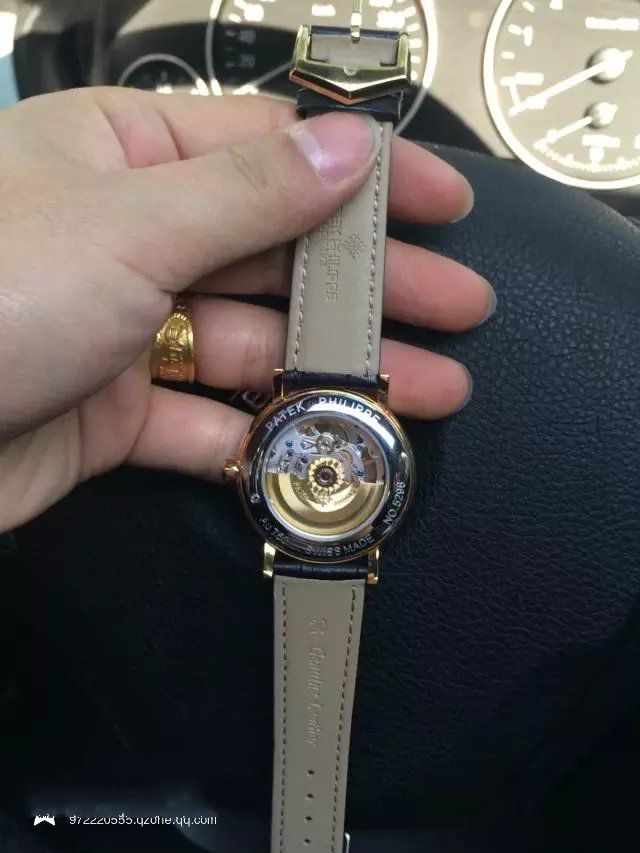In the photograph, a hand with a gold ring on the ring finger is prominently holding a Patek Philippe watch with a light gray leather band. The watch has a transparent case, revealing its intricate gears and inner workings, and bears the inscriptions "Swiss Made" and what appears to be a serial number, partially readable as "number 59...6." The hand, likely male due to its larger size and overall appearance, is positioned against the backdrop of a car's interior. This includes visible speedometer and tachometer dials, which are light gray with white markings against a darker background possibly indicating the dashboard and seats. At the bottom of the image, there is white text that seems to be a web address, although it is somewhat obscured and difficult to read.